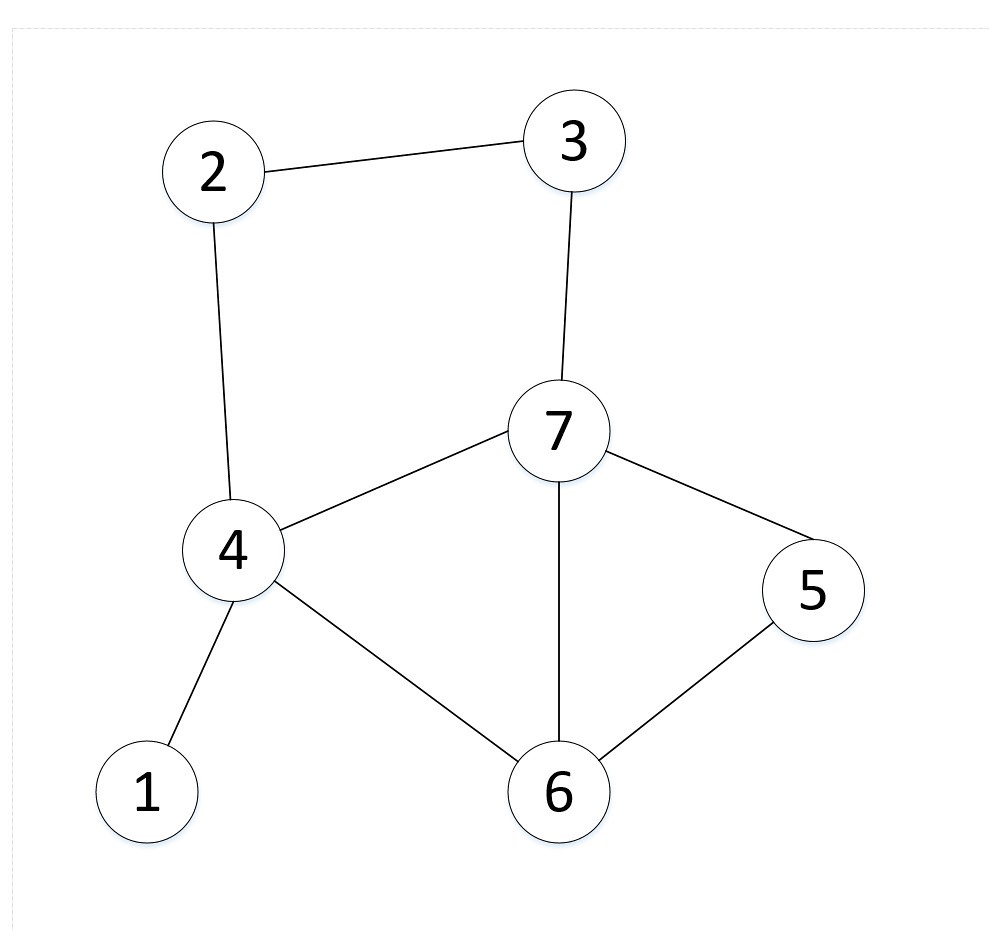This image appears to have been generated using a computer program, and it resembles the kind of diagram found in textbooks or educational handouts. 

Starting from the upper left corner, about three inches to the right, there is a circle marked with the number "2" in black text. A thin black line extends approximately four inches from this circle, connecting to another circle containing the number "3".

Following a downward line of about three inches, we reach a circle labeled with the number "7". From here, a diagonal line to the left leads to a circle with the number "4". Extending to the left from the number "4" is another line that reaches a circle containing the number "1".

Conversely, a line to the right of the number "4" extends all the way down to a circle at the bottom, labeled with the number "6". From here, moving diagonally up and to the right, a line connects to a circle containing the number "5".

The number "5" circle has a line coming out from its top center, extending to the left, which then reconnects to the number "7" circle.